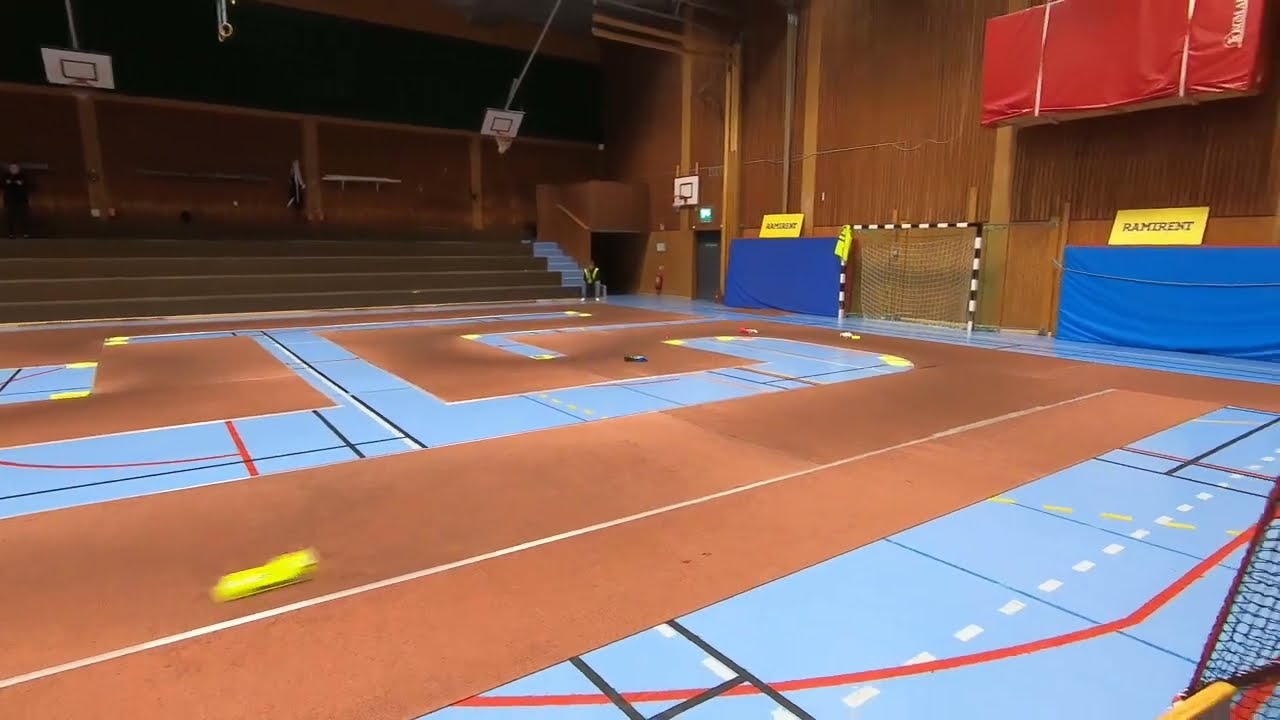The photograph depicts an indoor gymnasium with prominently brown wooden walls on the left side of the image and extending towards the center. Several brown-colored bleacher structures are positioned along this side, upon one of which a solitary person is seen sitting near a doorway. The gym floor features a mix of dark tan brown and light blue areas, intricately patterned with various colored lines including red, white, black, and yellow, likely delineating different game zones.

Large blue mats are arrayed upright against the center and right wall, crowned with yellow signs bearing white writing that reads "RAMIRENT." Between these mats sits a black and white striped net, possibly for indoor soccer, with striped poles supporting it. Additionally, a large red gymnastics mat is hoisted in the top right corner, secured by straps. Basketball hoops are retracted toward the ceiling, above the bleachers, showcasing white backboards with yellow designs. The overall scene hints at versatile usage, potentially including a track for remote-controlled cars, speculated from the unique court layout and the presence of the person possibly operating a remote control.